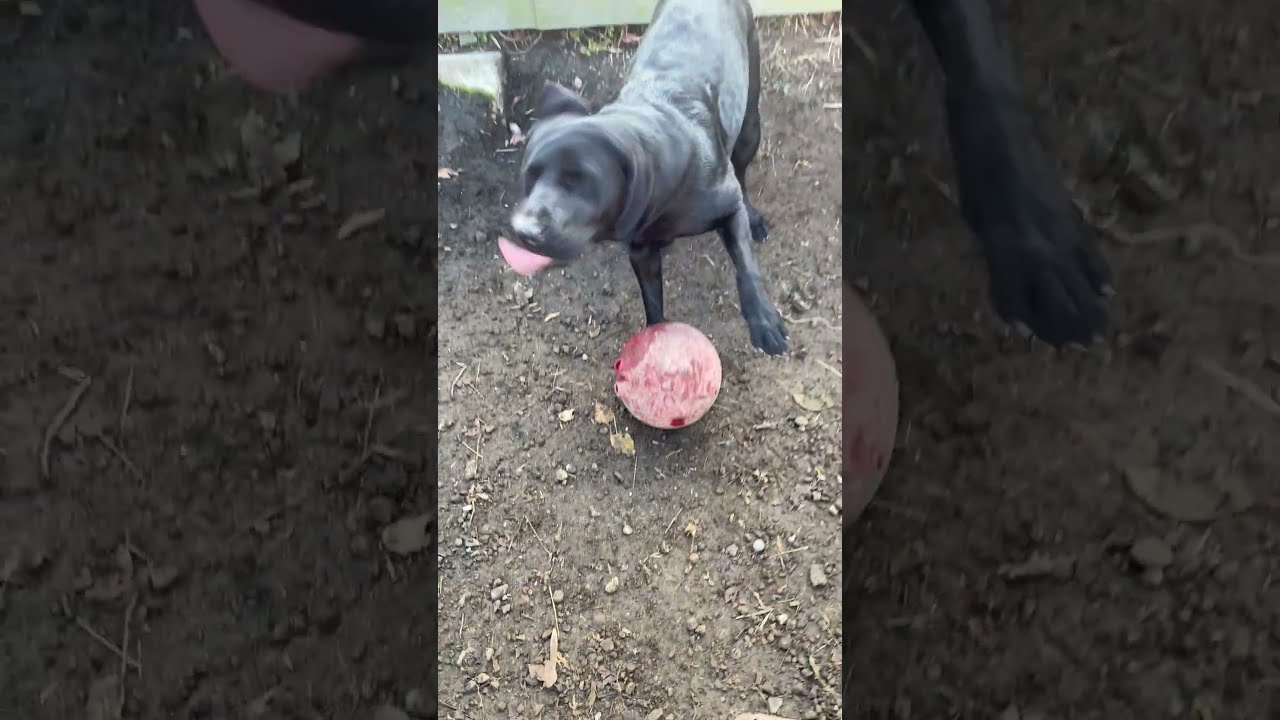This outdoor photograph captures a lively black dog with short fur and a pink tongue hanging out as it plays with a worn, dirty red ball. The dog stands on a dry, brown soil yard scattered with brown dried leaves, with no grass in sight. Its left front paw is raised, and its right paw is positioned near the ball, giving the impression that the dog is in mid-motion, possibly shaking its head as one ear is perked up while the other curls around its head. The sun shines brightly, casting a warm light on the scene. In the background, the upper left corner features a gray rock or partially buried brick, contributing to the rustic feel of the setting. The image is the center panel of a triptych, with the focus sharply on the dog and ball while the left and right panels are blurred out. There is no text on the photo.